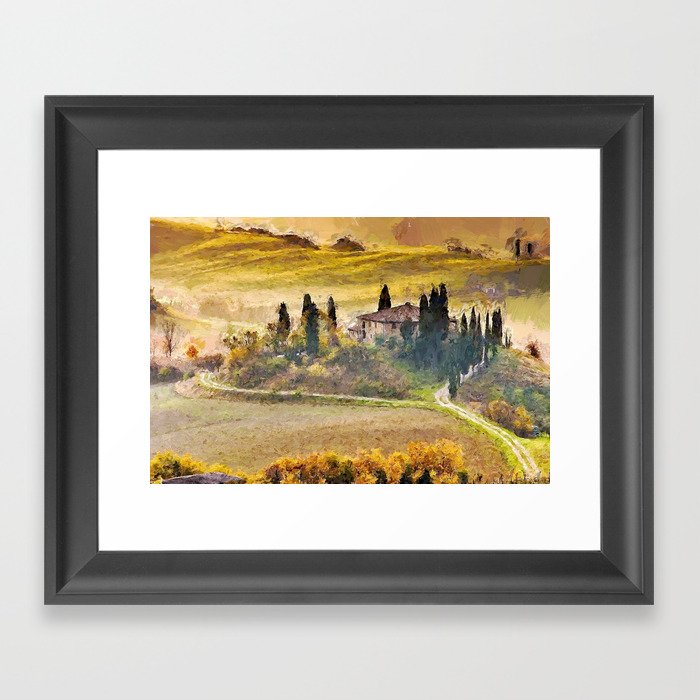The image showcases a computer-generated, photorealistic painting encased in a simple, black rectangular frame with a thick border. This frame is set against a plain gray backdrop. The artwork within the frame depicts a tranquil pastoral countryside scene. At the center is a light brown or beige house with a darker brown, triangular roof. Surrounding the house are tall, dark green trees, notably lining a gravel driveway on the right side, which winds its way around the property. The landscape features a mixture of yellow, light green, and brown foliage, indicative of farmland. There are rolling hills in the background, painted in lighter green shades, adding depth to the scene. The painting is bordered by a white mat, enhancing its vivid and serene depiction of rural life.